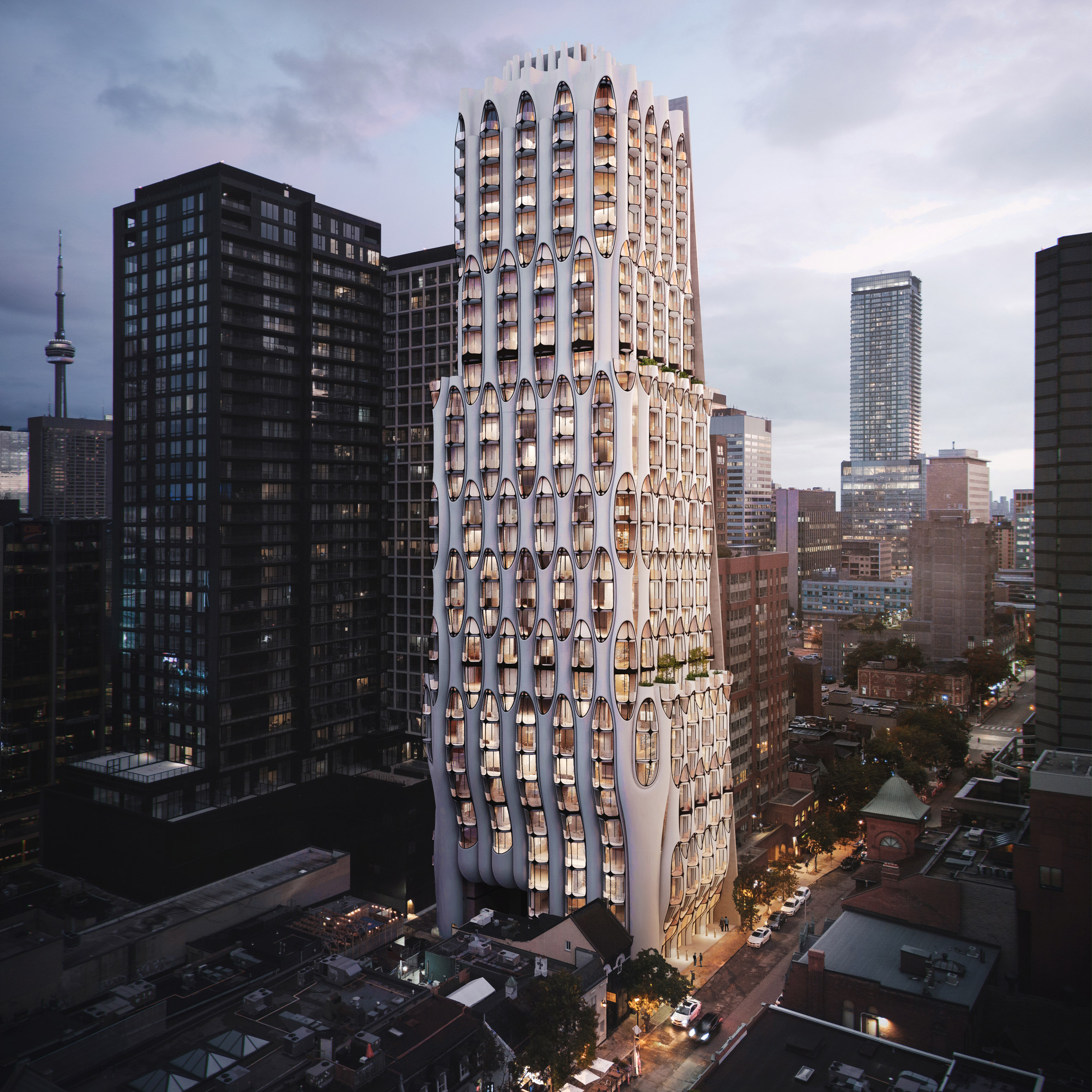The image depicts a striking modern skyscraper set in a dense urban downtown area. This white and gold building features a distinctive, futuristic design with numerous windows. The unique architecture includes wavy lines that ascend its height and oval shapes that adorn the façade from top to bottom. These ovals house balconies and add a distinctive round curvature to the building's overall look. The base of the building has a wavy design, reminiscent of Gaudi's architectural style in Barcelona. Surrounding the main structure are other tall buildings, including a sleek black rectangular building to the left and a thin tower with a circular restaurant halfway up. The scene is set against a hazy sky with darker blue hues and thin dark clouds, adding to the contrast. At street level, a few cars are parked, accentuating the bustling downtown setting.